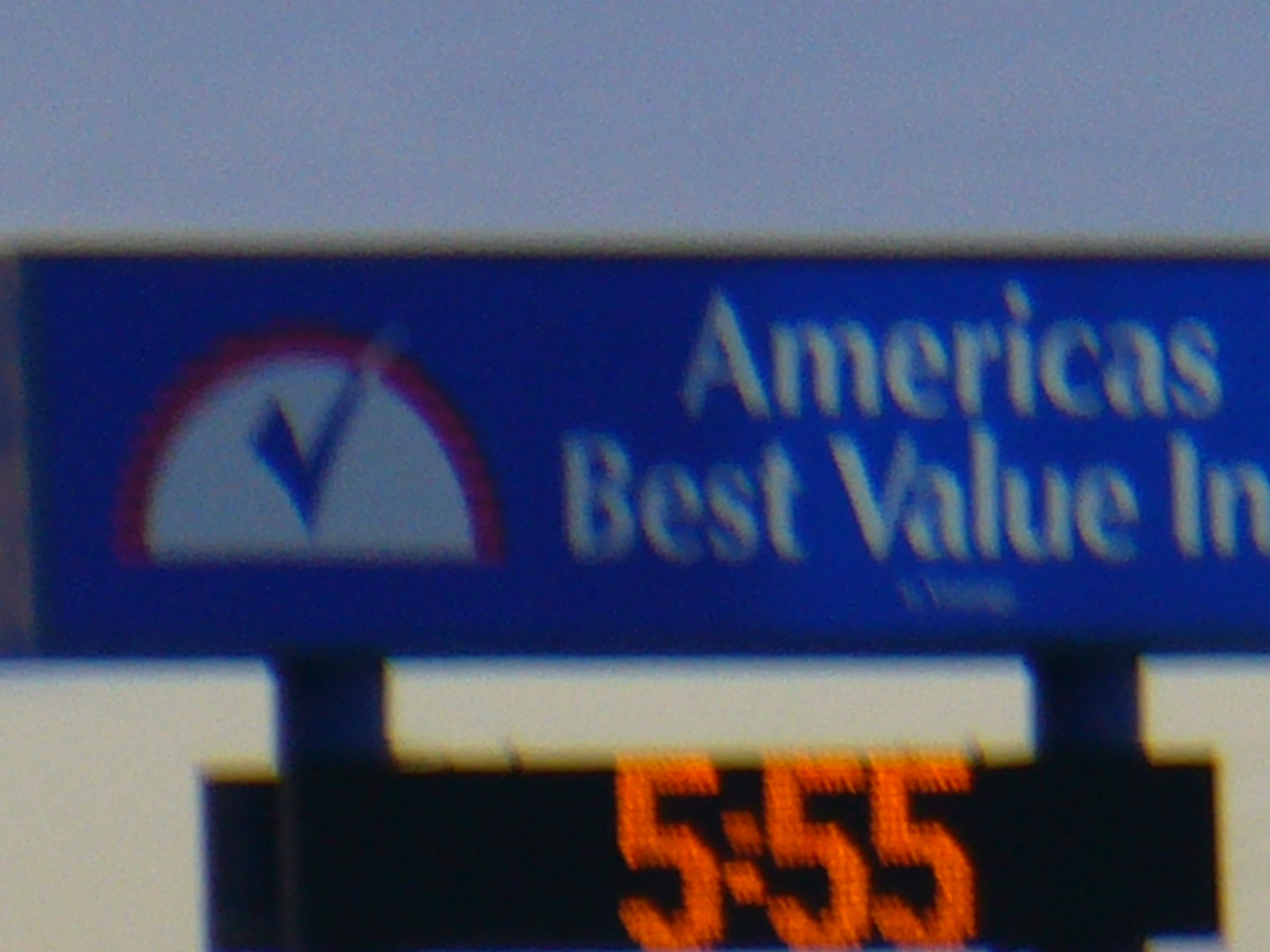This image depicts a large, rectangular business sign for “America's Best Value Inn.” The photograph appears to be taken outdoors and is notably blurry and zoomed in, likely causing some of the distortion. The sign itself is blue with white text, stating "America's Best Value Inn." The top part of the sign features a logo with a blue check mark inside a semicircle. The semicircle has a white background and an outer red stripe. Below the main sign, a digital clock with bright red numbers on a black background displays the time "5:55." The photograph's background shows a gray, grainy sky with a hint of yellow near the horizon, suggesting early morning or late evening. The bottom of the photo cuts off at the bottom of the digital clock.